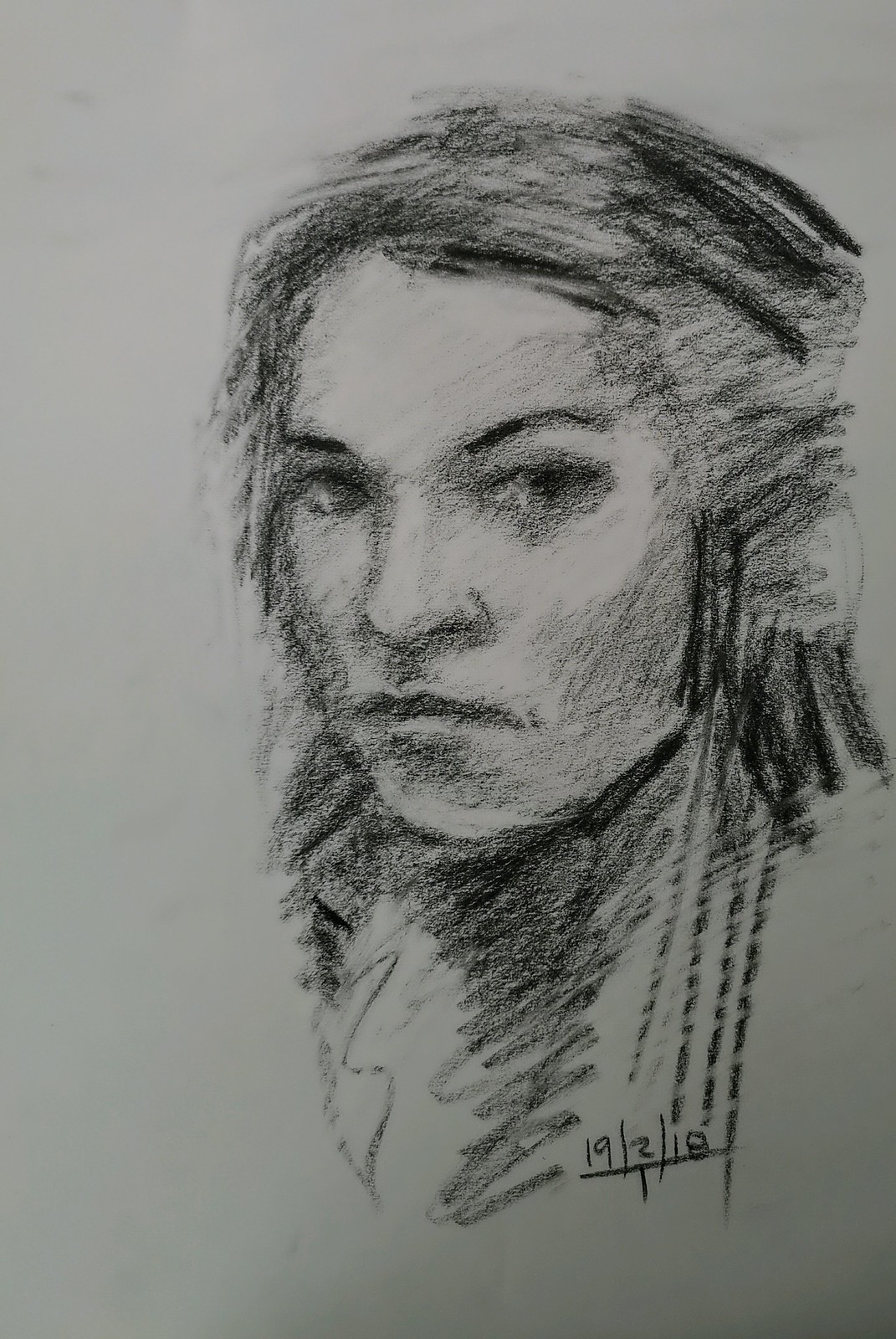This captivating charcoal sketch features an elegantly drawn woman who occupies nearly the entire page, positioned slightly to the right. Her gaze is directed just over the observer's left shoulder, lending an intimate feel to the composition. The artwork is dated with a European-style inscription, "19-3-18," which translates to "3-19-18" in the US date format. Despite its seemingly quick execution, the artist has skillfully achieved remarkable shading and depth, creating a compelling and well-executed portrait.